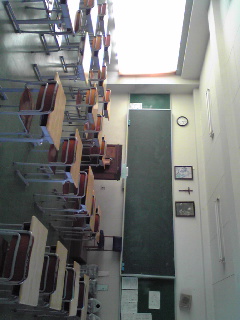The image depicts a classroom setting with numerous wooden desks featuring tan tops and built-in storage compartments underneath. At the front of the classroom, a long rectangular chalkboard stretches across the wall, serving as the focal teaching area. Above the chalkboard hangs a round clock with a black frame, keeping time for the students and teacher. Additionally, the wall above the chalkboard is adorned with two pictures, flanking a cross positioned centrally between them. The overall scene captures a traditional and organized learning environment.